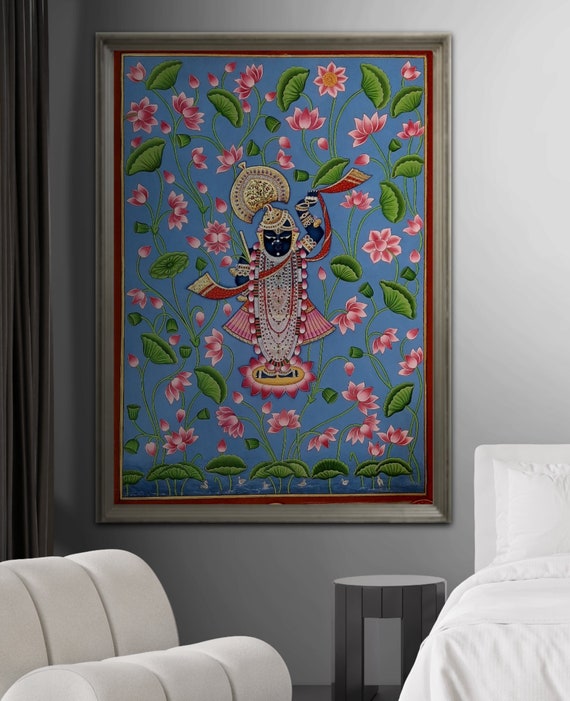In the image, we see a cozy bedroom corner adorned with a striking piece of art. The bottom right of the frame captures a sliver of a white bed, complete with a white headboard, pillow, and pristine bed linen. Adjacent to the bed, on the left side, stands a gray, stool-like night table complemented by a couple of white cushions and flanked by a vertical gray curtain. The background of the image features a gray wall, setting a calm and neutral tone for the room.

Dominating the wall is a beautifully framed painting with a silver-gray outer frame and a narrow dark red inner border. The artwork itself is vibrant, featuring a light blue background adorned with green leaves, lotus flowers, and pink blossoms. At the center of the painting is a detailed depiction of an Asian deity, identifiable by its fan-shaped headdress. The deity showcases an intricate design with a beige figure, a black face, and a red scarf cascading around it. The figure also has yellow, white, and gray elements that add to its ornate appearance. This mix of botanical elements and a historically significant statue creates a captivating focal point in the room.